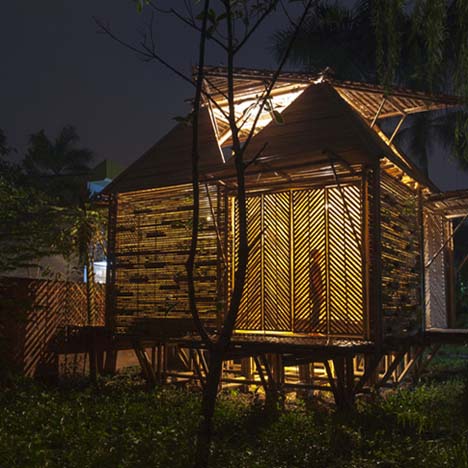The photograph captures a nighttime scene featuring two elevated hut-like structures in a yard, with one prominently illuminated from the inside. These structures are made predominantly of wood and bamboo, with intricate diagonal slats on the walls that allow glimpses of a person standing inside, facing right and looking upwards towards the light source. Their triangular roofs are designed to open and close with flaps, which helps with ventilation, and the huts are supported by wooden legs that raise them about a foot above the ground. In the backdrop, a fence encloses the yard, and a young tree is visible in the foreground. Above, a star-studded night sky adds an ethereal touch to the scene.